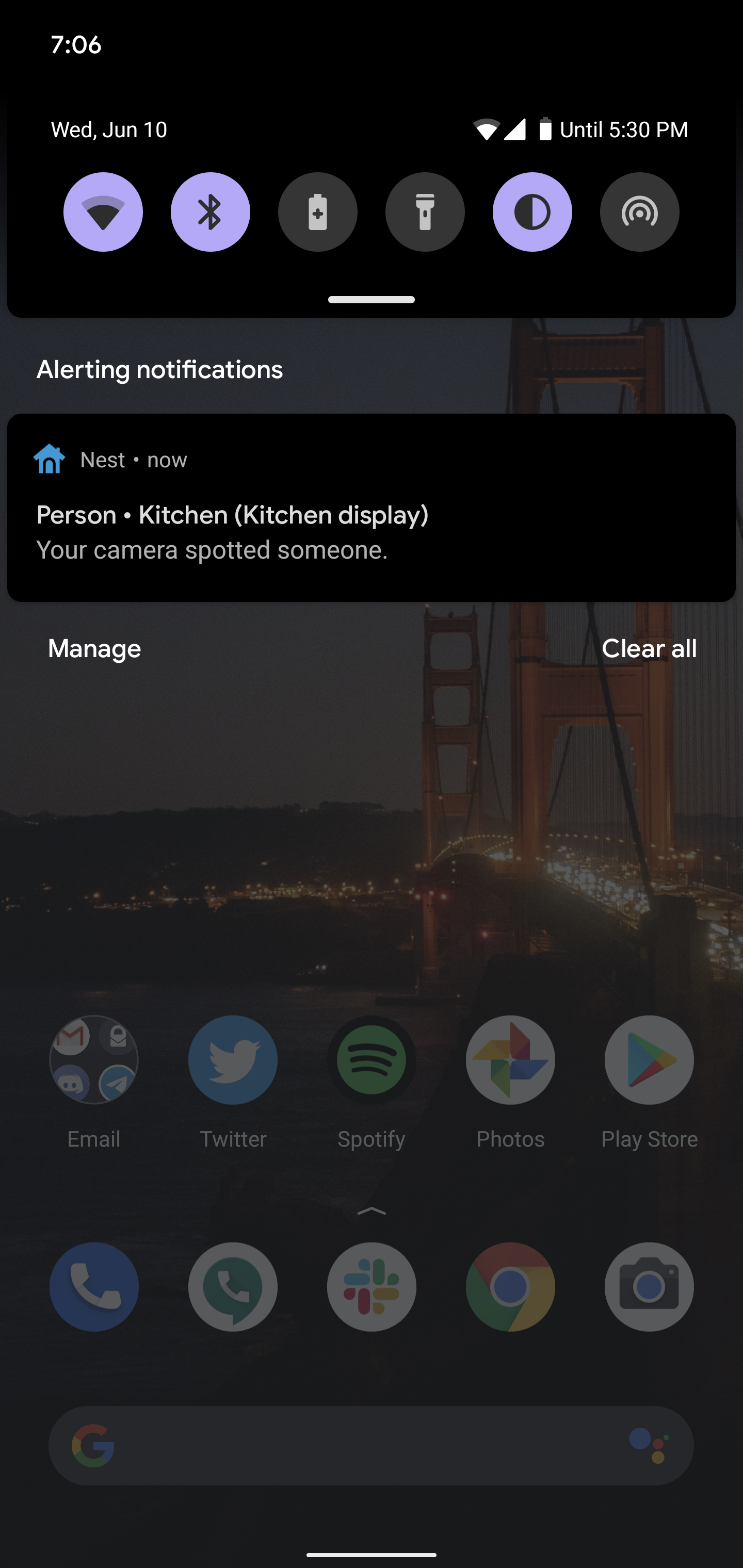This is a detailed screenshot from a cell phone, primarily characterized by a nearly black background with light purple highlights. Located in the upper left corner, the time and date are clearly displayed as 7:06 PM, Wednesday, June 10th, alongside a battery icon that shows the battery is either nearly full or fully charged. Below this, the display shows a typical swipe-down menu for accessing quick settings.

Highlighted in purple are the Wi-Fi and Bluetooth buttons, indicating these features are active. Dimmed and unselected are the battery and flashlight buttons. The brightness button is highlighted in purple, signifying its active status. The final button in this row is unclear in its function but remains unselected.

Below these buttons, a bar labeled "Alerting Notifications" shows a recent alert from Nest, indicating a person has been spotted in the kitchen by the kitchen display camera. Accompanying this notification, a bandage icon is situated to the left and a "Clear All" button is on the right.

The phone's wallpaper features a stunning night-time image of the Golden Gate Bridge, illuminated with the lights from vehicular traffic crisply visible. Underneath this beautiful overlay, various app icons populate the homepage, including Twitter, Spotify, Google Photos, Google Play Store, the phone launcher, WhatsApp, Google Chrome, and the camera app, among others.